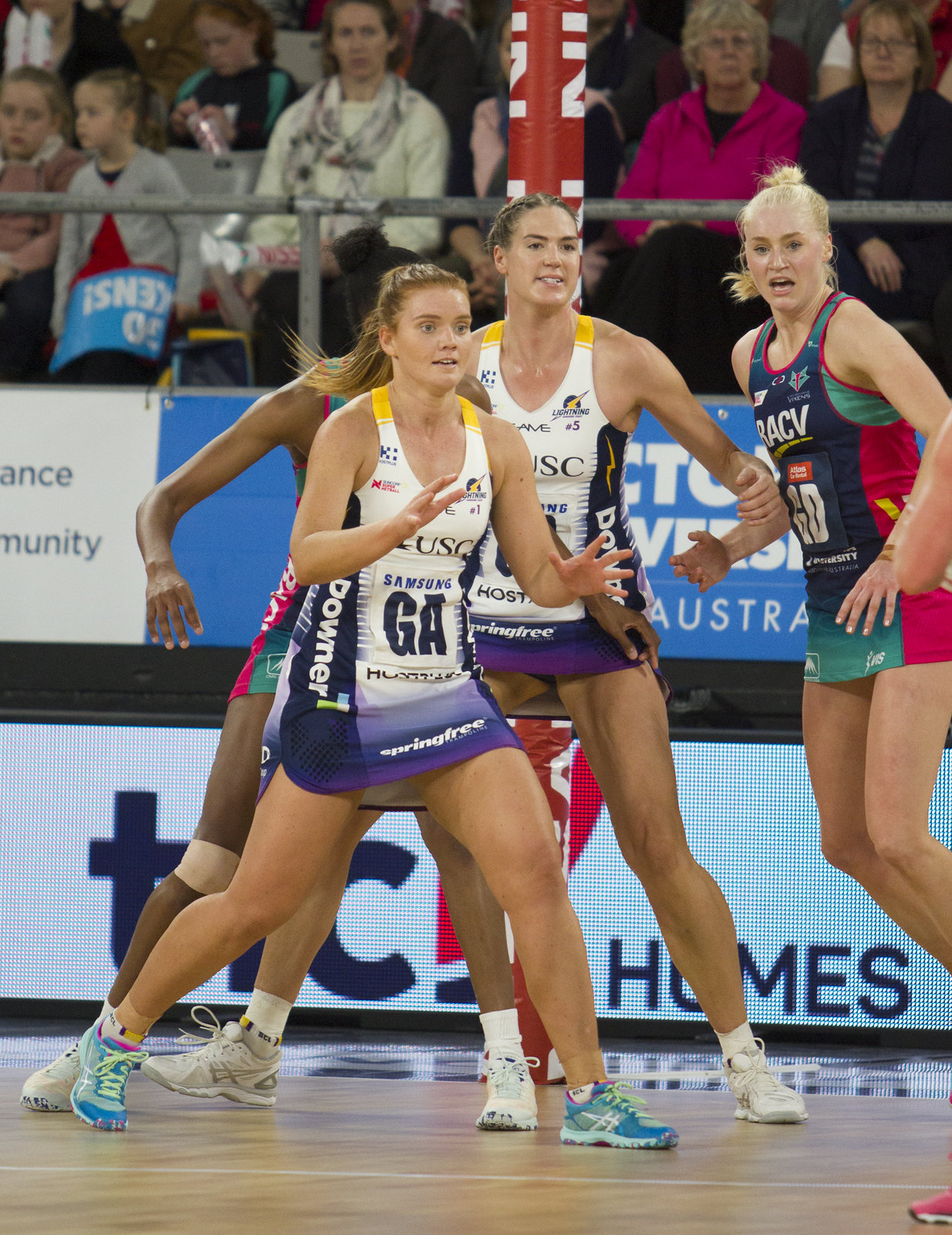The photograph captures an intense moment at a women’s volleyball match played on a light brown wooden court marked with white lines. Central to the image are four female players in sleeveless jerseys that extend to about their calves. The team in purple and white, with distinct white lettering, is facing the team in green and red, also with white text. 

Prominently featured in the foreground, a Caucasian player with light brown hair pulled back is moving energetically to her right, arms bent and extended as if poised to catch a ball. Her uniform is a white tunic with dark blue side striping and dark blue lettering across the front, and she wears light blue athletic shoes with no socks. Beside her, another player from the same team, also in motion, has darker hair pulled back and supports her teammate's efforts. She sports white athletic shoes and white socks. 

Opposing them, a tall, very blonde Caucasian player in a black tunic with red vertical side stripes and white text on the front appears to be jumping, with her knees bent and arms bent but not extended. In the background, the audience sits on gray-colored seats, separated from the court by a metal railing. The crowd includes a young child and what appears to be their mother, a woman in a pink hoodie, and another woman with dark hair and glasses. One player's shirt features the letters "GA," possibly indicating Georgia, and there are additional visible logos and text, such as "RACV" and "USC," on the players' uniforms. The overall atmosphere is charged, with the focus on the players and the anticipation of the crowd palpable.